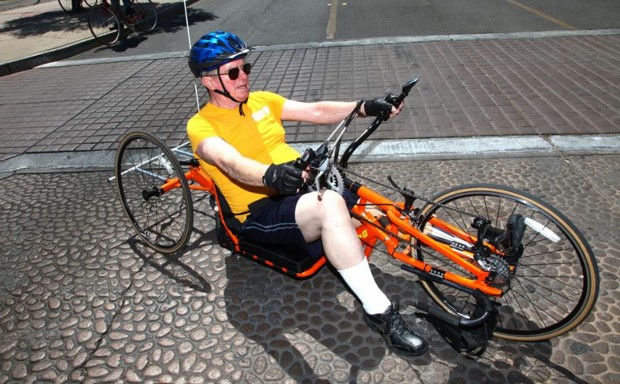In this image, an elderly white man, likely in his 60s or 70s, is captured sitting on a unique three-wheeled recumbent bicycle. The bike features an orange frame with one wheel in the front and two in the back, complete with a backrest and a small carrier case attached at the rear. The man, dressed in a yellow t-shirt, black shorts, white socks that run up his shins, and black sneakers, is poised for a ride. He's equipped with black sunglasses, black gloves, and a dark blue helmet. His bike is parked on a pebbled ground surface, with a stone path and street nearby, suggesting an outdoor urban setting. The man appears to be getting ready to start, with his hands gripping the black handlebars and his mouth slightly open.